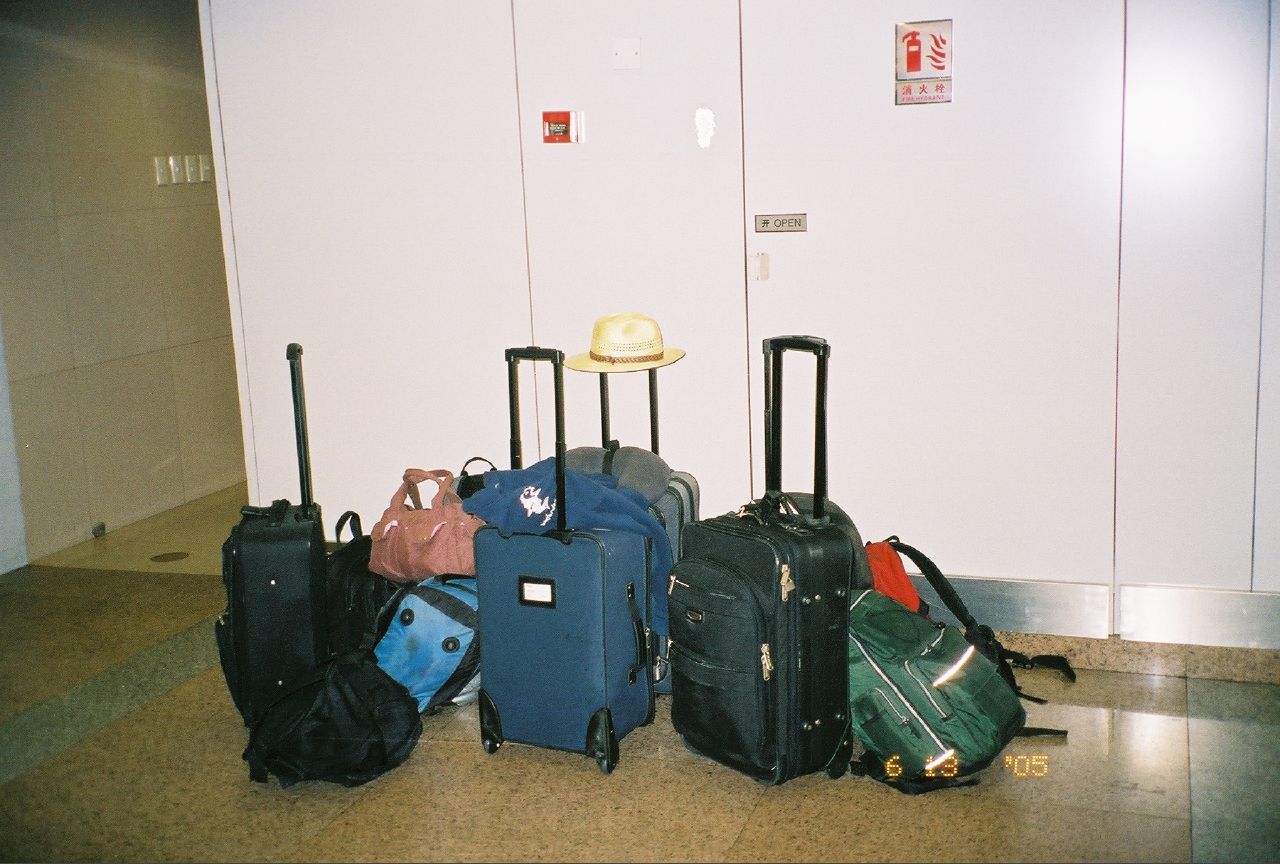The image depicts a cluster of luggage positioned on a tiled floor, possibly in an airport terminal or near the entrance to a restroom. The wall behind the luggage is white, adorned with signs featuring characters in red, likely Chinese, Japanese, or Korean. The collection includes various types and colors of luggage, specifically featuring rolling carry-on suitcases and non-wheeled bags. Prominently, a green backpack is positioned to the right, followed by a gray piece of carry-on luggage with a straw hat on its extended handle. A blue carry-on suitcase with a blue sweatshirt draped over it is also notable. Additionally, there are several other pieces: at least one more black suitcase turned left with its handle extended, and a few duffel bags and soft-shell bags completing the assortment. The scene is set in front of a panel zone that includes fire extinguishers, indicated by symbols on the wall.